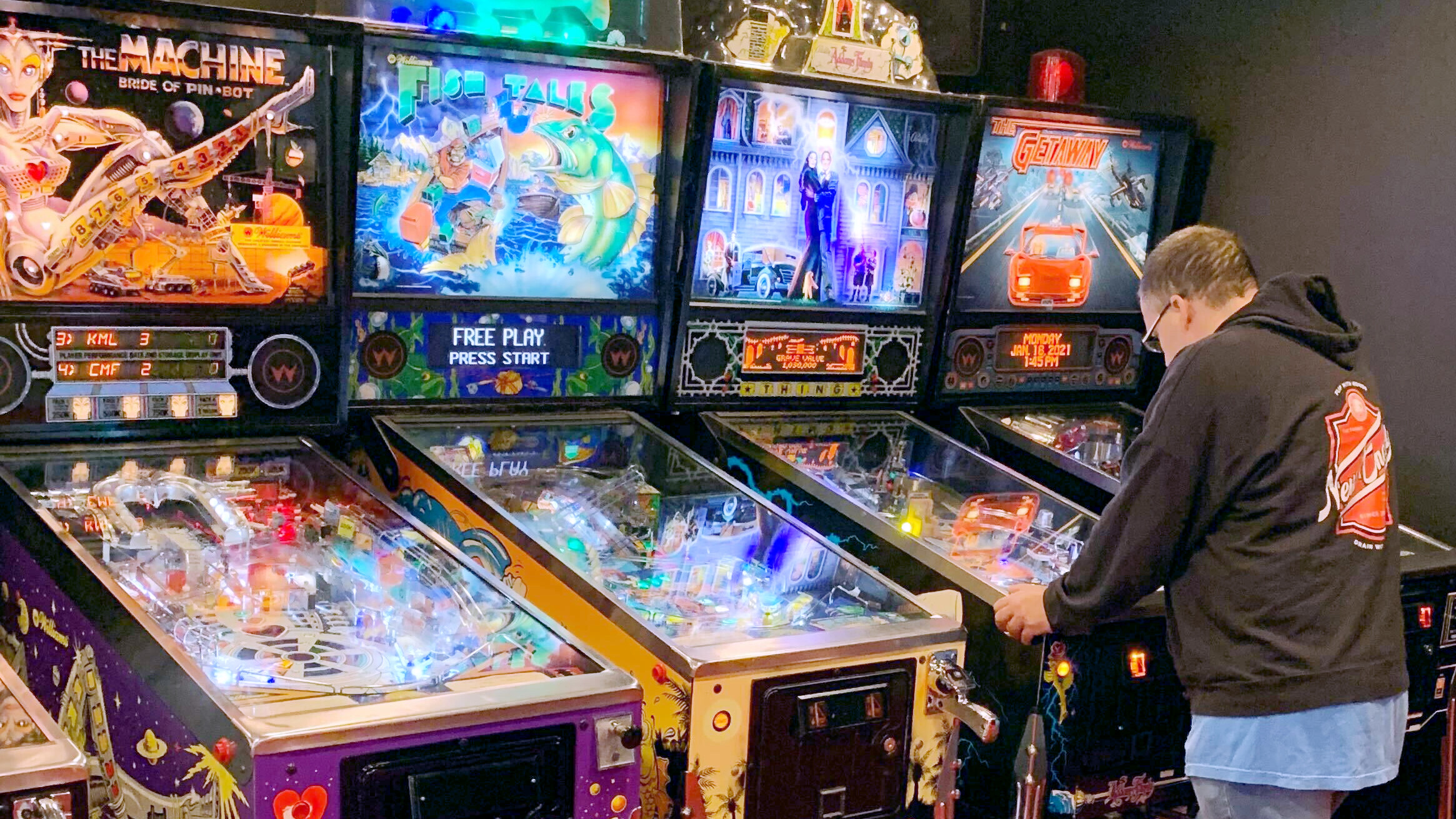This landscape-mode photograph captures an arcade scene featuring four vividly-lit pinball machines with a glimpse of a fifth. From left to right, the pinball machines are "The Machine: Bride of Pinbot," "Fish Tales," "The Addams Family," and "Getaway," each adorned with brightly colored lights, including some illuminated headers. The locale has dark gray walls which provide a contrasting backdrop to the vibrant pinball machines. A middle-aged, heavy-set white man, wearing a black hoodie with "North Newcastle" on the back, a blue t-shirt, and jeans, stands intently playing "The Addams Family" pinball machine. He wears glasses and has his head down, engrossed in the game. On the far right, the "Getaway" pinball machine is distinguishable by an image of a Ferrari.